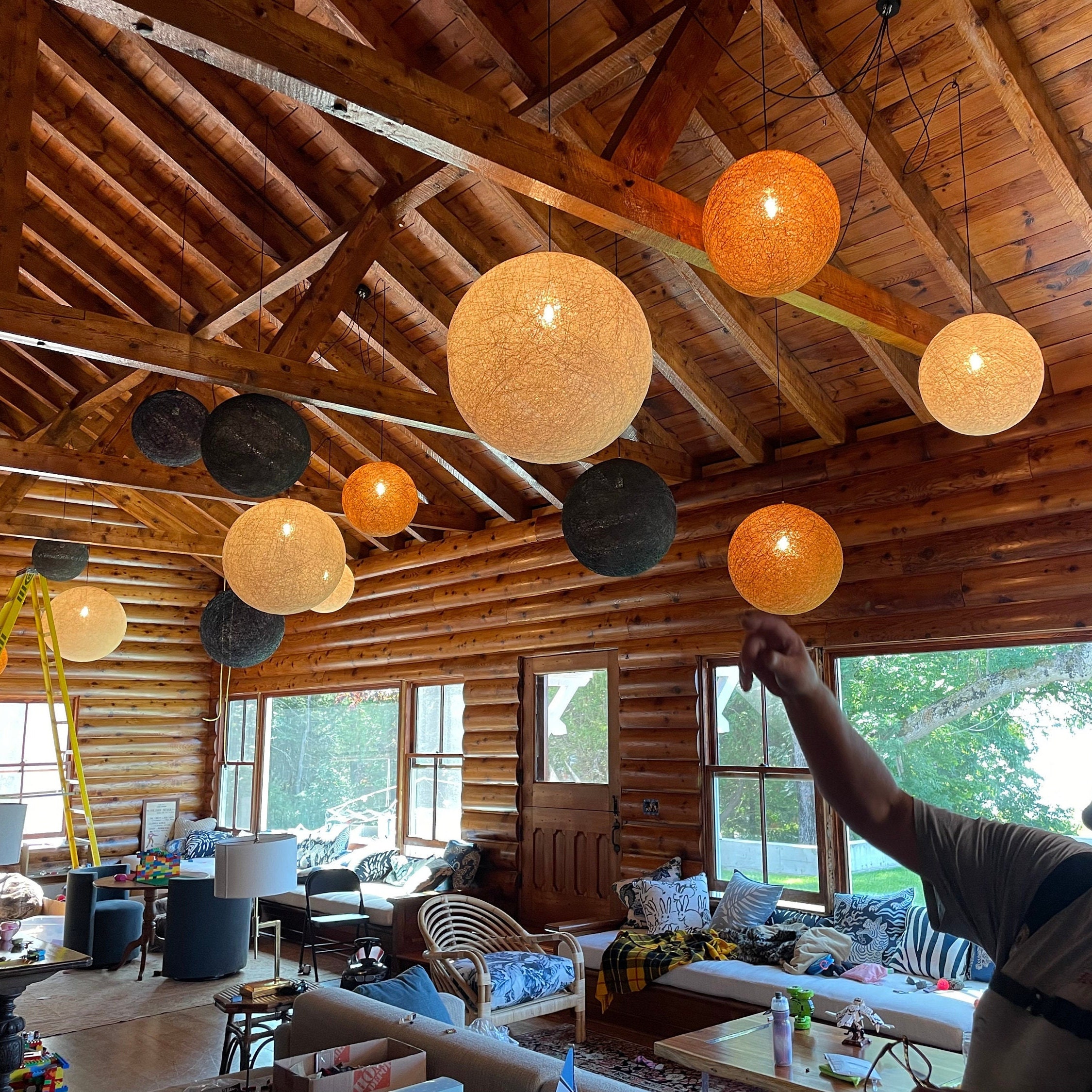A captivating photograph taken from within a cozy log cabin showcases a unique interior lighting display. The rustic charm of the cabin is highlighted by the visible logs used in the walls, and an open ceiling featuring wooden beams and planks adds to the ambiance. From the ceiling, sturdy black cables descend, each supporting a light bulb encased in a semi-transparent sphere. These hanging orbs create a mesmerizing effect, with their gentle illumination in varying hues - some glowing with a light peach color, others emanating a deeper orange, and a few appearing almost black, offering a striking contrast. The result is a ceiling adorned with a constellation of glowing orbs that enhance the warm, inviting atmosphere of the space.